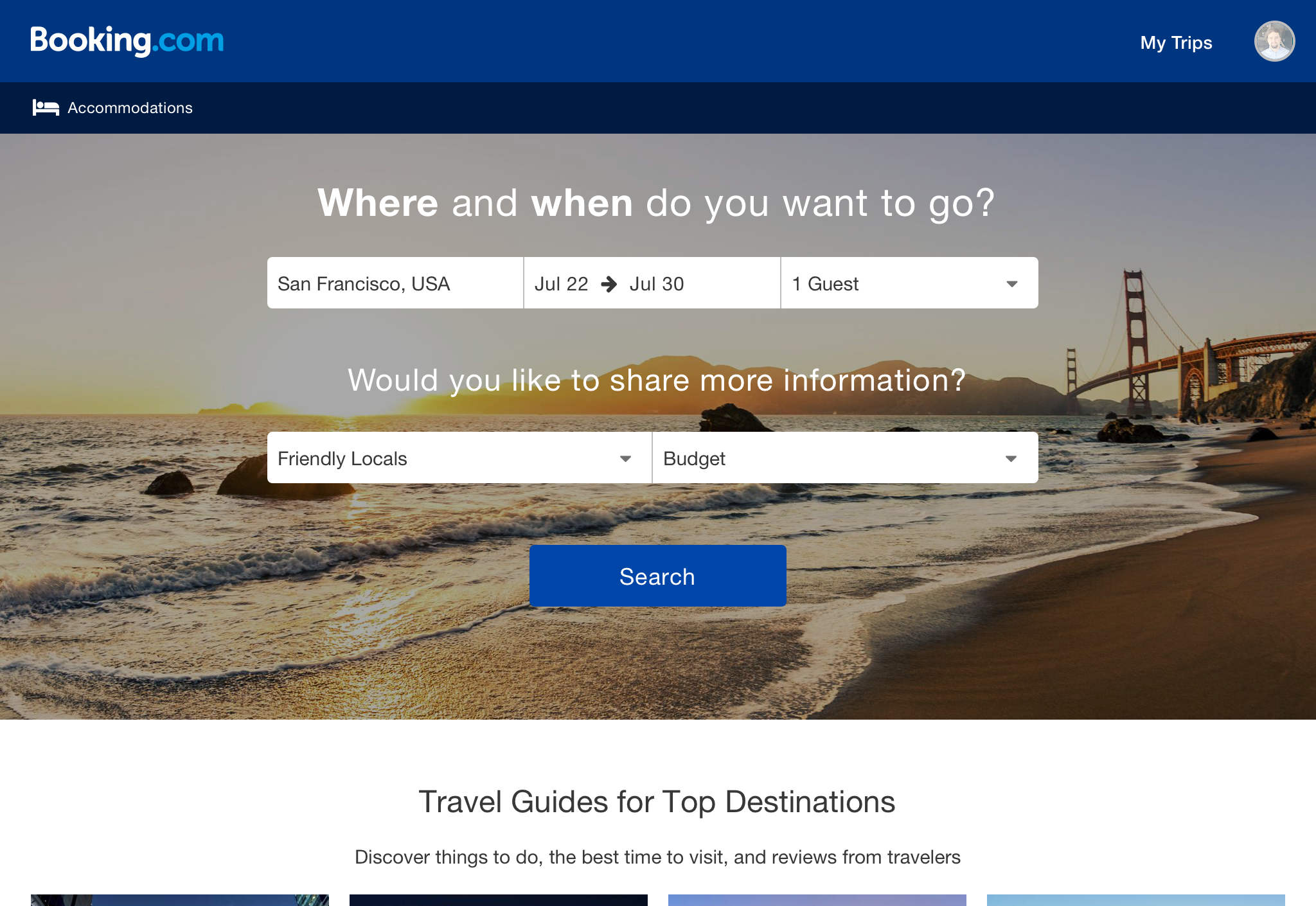In this screenshot of the Booking.com website, the header is prominently set against a blue background. On the upper left corner, the "Booking.com" logo is displayed, with "Booking" in bold white text, and ".com" in bold blue text. On the upper right section of the header, there is a menu item labeled "My Trips," which is accompanied by an icon of a person's face.

Directly beneath this header is a black banner featuring a white icon of a bed with a person sleeping on it. Next to this icon, the text "Accommodations" is displayed in white.

The main background image of the website showcases a scenic photo. Starting from the center right, a bridge appears and leads towards a mountainous area. The image also captures the lower right corner, where a beautiful beach with waves crashing onto the shore can be seen, complete with the white foam of the waves as they meet the ground.

At the center top of the image, the website's search prompt reads, "Where and when do you want to go?" Underneath this prompt are three search boxes aligned horizontally: the first box specifies the location, "San Francisco, USA"; the second box indicates the travel dates, "July 22nd to July 30th"; and the third box is a drop-down menu that reads, "1 guest."